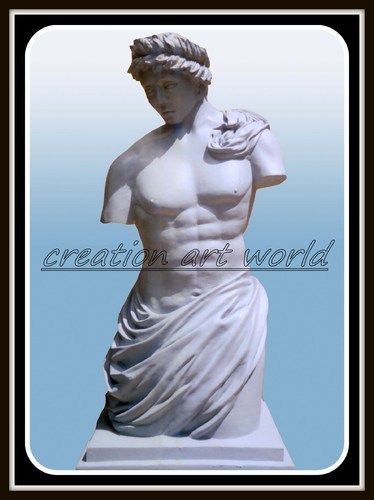The image features a detailed statue reminiscent of the Venus de Milo, depicting a man with his arms cut off, adorned in minimal clothing. The man, donning a folded headscarf and a cloth wrap from his waist to his thighs, is gazing thoughtfully towards the bottom left. On his left shoulder, a towel is draped. This statue sits elegantly on a white pedestal and is framed in black, gray, and white. The background gradient transitions from white at the top to light blue at the bottom. Over the statue, the text "Creation Art World" is prominently displayed, serving as a watermark. The overall color palette includes shades of black, gray, white, and various tones of light blue, enhancing the classic aesthetic of the artwork.